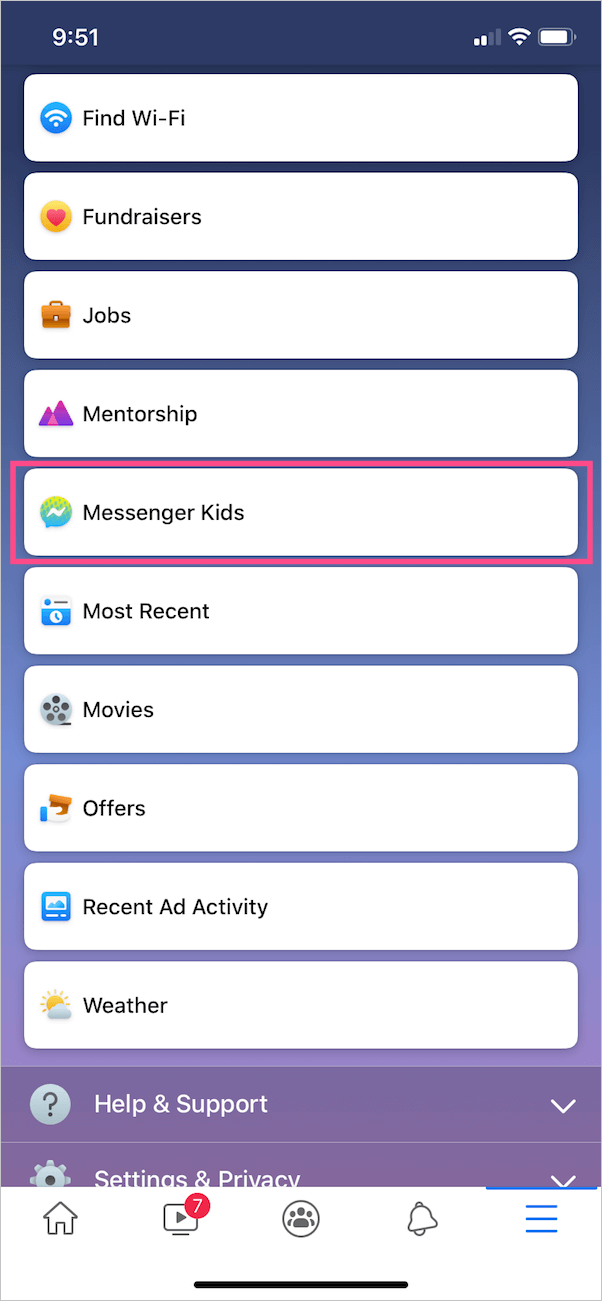The screenshot depicts a mobile phone interface showcasing a menu with various options. The top of the screen displays a partial search input "951" above options including "Find Wi-Fi," "Fundraisers," "Jobs," "Mentorship," and "Messenger Kids." A prominent red rectangle highlights the "Messenger Kids" option. Additional options visible in the menu include "Most Recent," "Movies," "Offers," "Recent Ad Activity," and "Weather."

The background gradient transitions from a deep blue at the top to a purple hue towards the bottom. The lower portion of the screen features a navigation bar with icons: a home button, a video-related icon similar to YouTube's, a friends or contacts icon, a notification bell, and a blue-colored hamburger menu.

The bottom section also includes options for "Help and Support" and "Settings and Privacy." The interface appears to be part of a social media or service application, with an organized and colorful layout.

This detailed snapshot provides a comprehensive overview of the phone's current screen and navigational points.